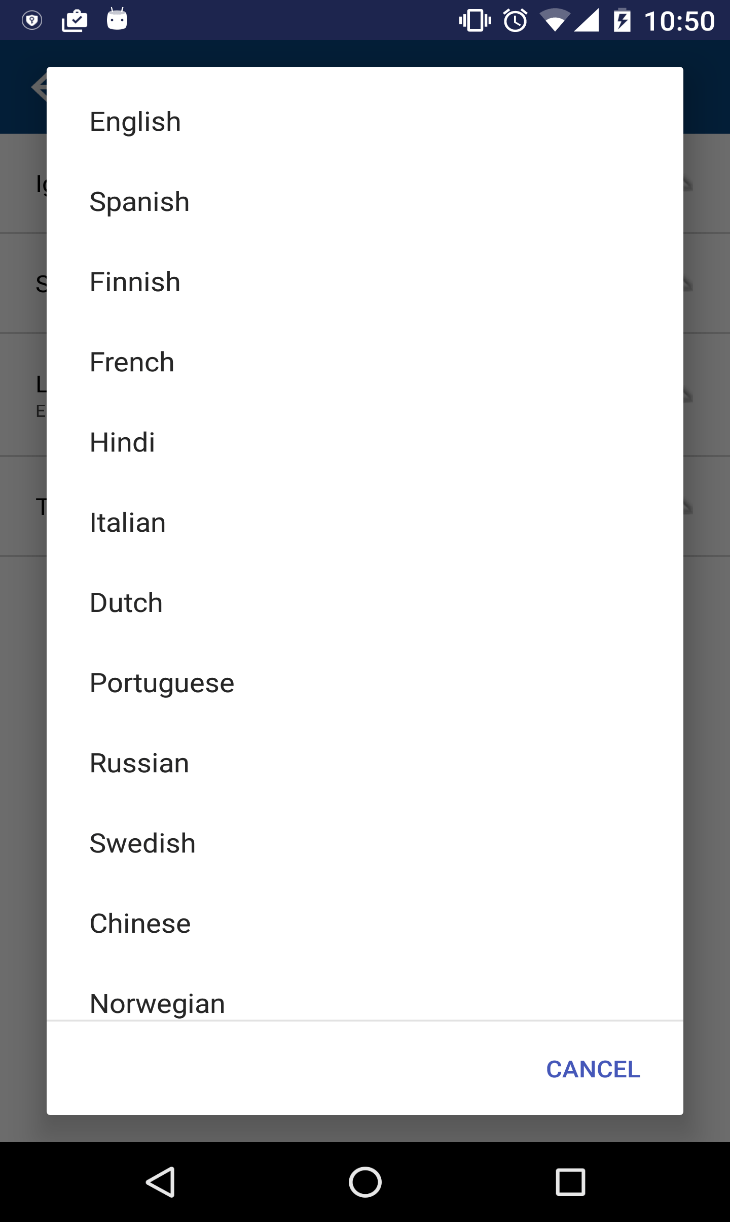This screenshot, captured from an Android mobile phone, features the language selection screen during initial setup or within a specific application. The background is grayed out, providing contrast for the foreground elements. The top of the screen displays a row of indigo-colored icons, indicating various statuses: an Android icon, a vibrate mode indicator, an alarm clock icon, signal strength bars, a Wi-Fi icon, a battery meter, and the time displayed as 10:50, without specifying AM or PM.

Dominating the central 90% of the screenshot is a white screen adorned with black text, listing various language options: English, Spanish, Finnish, French, Hindi, Italian, Dutch, Portuguese, Russian, Swedish, Chinese, and Norwegian. Below these options, there is a blue text link labeled "Cancel."

At the bottom of the screen, a black navigation bar typical of Android OS displays three white icons: a back arrow, a circular home button, and a square for recent apps. These icons are essential for the device’s navigation. The screenshot is void of any other images or colors, focusing purely on the language selection options with no active selections made.